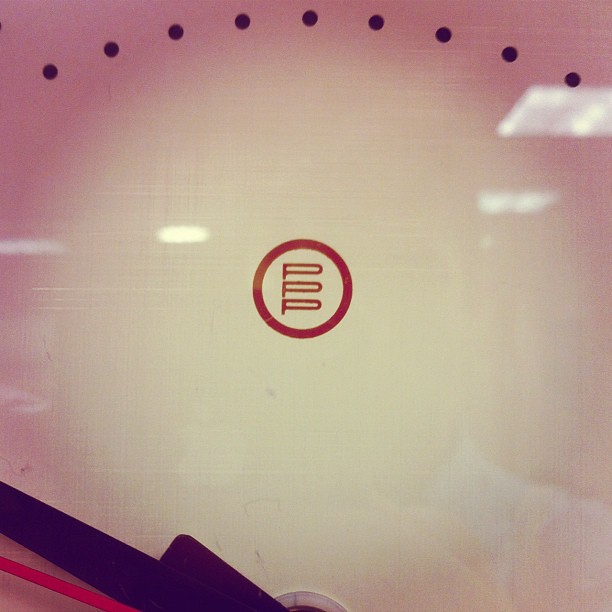The image features a gradient background transitioning from dark pinkish-purple at the edges to a creamy yellowish center. At the top of the image, there are nine small black circles arranged in a subtle arc. Dominating the center is a red-outlined circle. Inside this circle, three vertically-stacked symbols resembling elongated letters P with wide loops and curved ends on the right are positioned one above the other. Below these symbols, the lower portion of the image hints at clock hands, with a distinctively red second hand and a purple hand beneath it, suggesting the image may be a stylized or close-up section of a clock face.